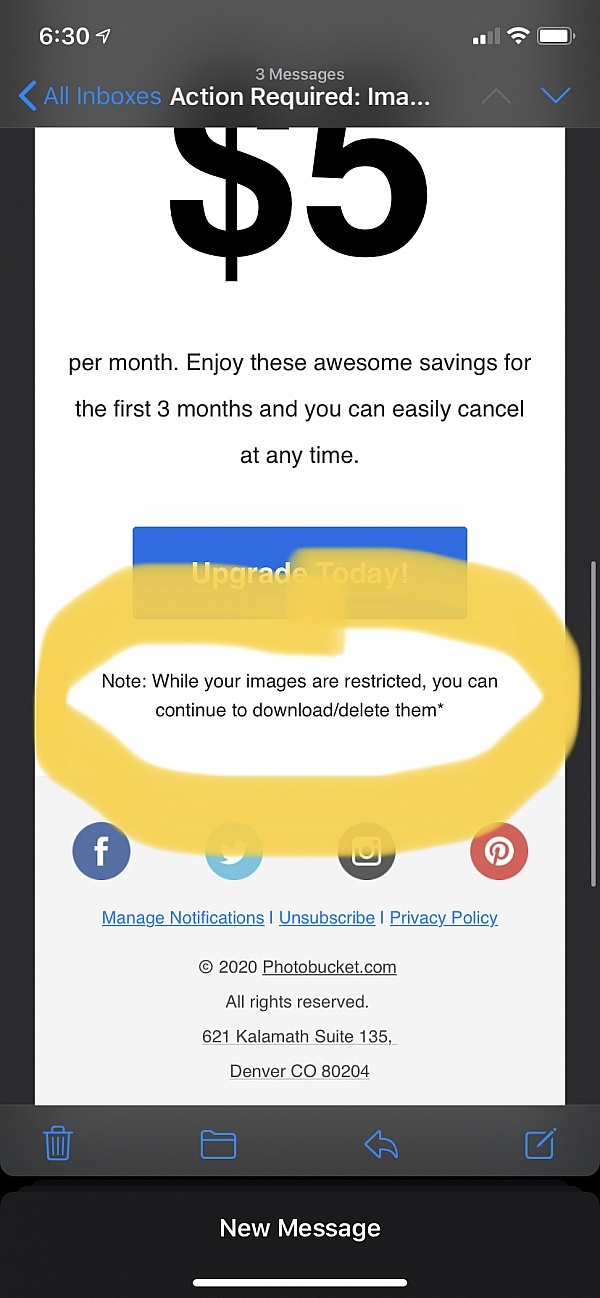The cell phone screen displays the time as 6:30 in the top left corner, while the top right corner showcases icons indicating strong cellular signal, Wi-Fi connectivity, and a fully charged battery. Centrally beneath the status bar, a notification reads "3 messages," followed by navigation instructions, with a left arrow icon and "All Inboxes" label. The main content area features a prominent message: "Action required. I am a..." and beneath this, in a white box, it offers a subscription deal - "$5 per month. Enjoy these awesome savings for the first three months. Easily cancel any time," accompanied by a bold "Upgrade Today" button.

Below the promotional message, a note appears: "While your images are restricted, you can continue to download or delete them." This note is highlighted with an imperfect, hand-drawn thick yellow circle, indicating it was marked manually rather than using a digital tool.

At the bottom of the screen, there are social media icons for Facebook, Twitter, Instagram, and Pinterest. Further below, options in blue underlined text include "Manage Notifications," "Unsubscribe," and "Privacy Policies." The footer displays the company's details: "2020 Photobucket.com. All Rights Reserved. 621 Kalamath Suite 135, Denver, Colorado 80204."

Finally, the bottom section includes icons for various functions: a trash can (delete), a folder (archive), a back arrow, and an edit tool. The very bottom indicates a "New Message" prompt.